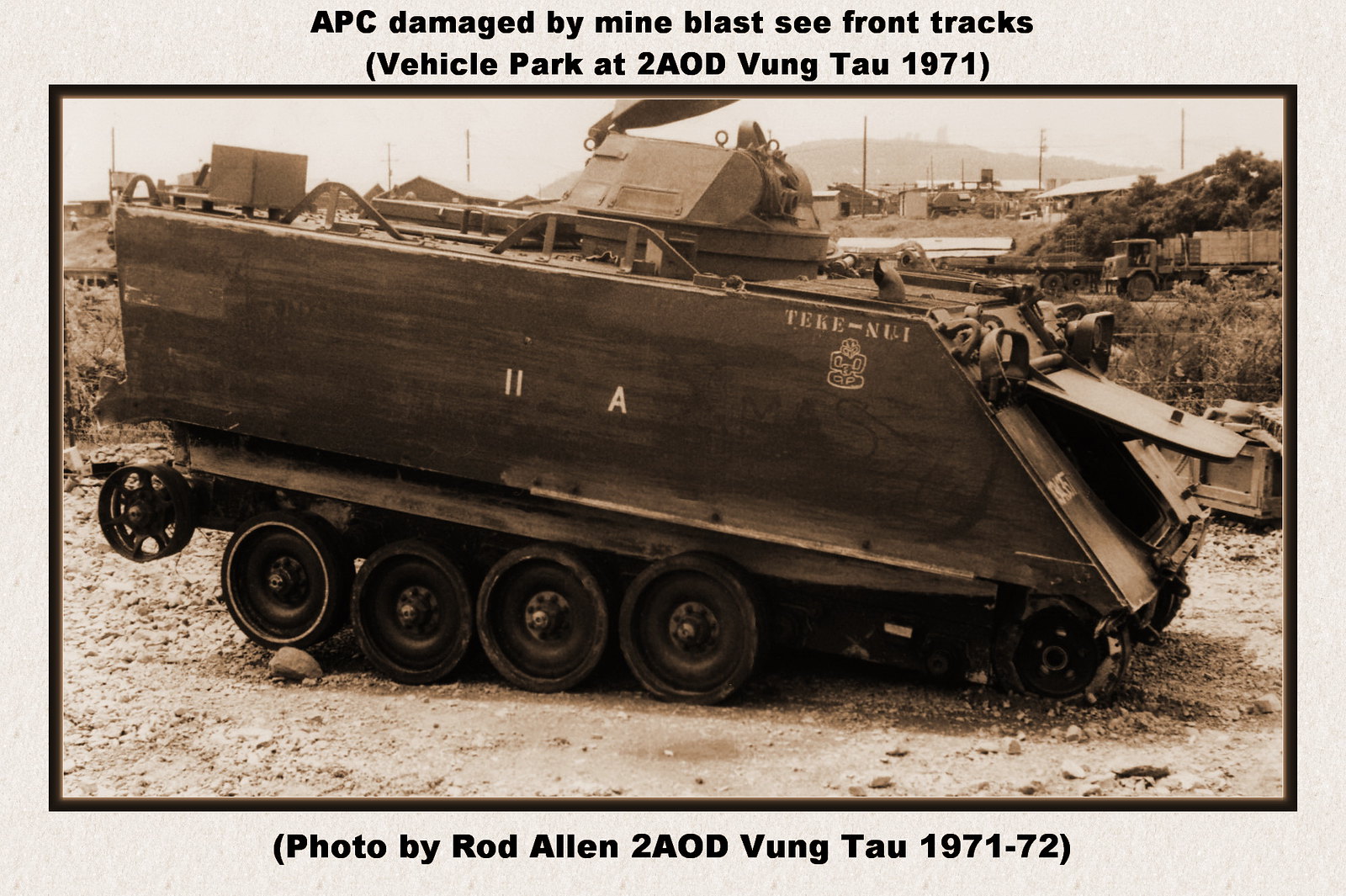This sepia-toned photograph, which appears to be from the early 1970s, captures an Army APC (Armored Personnel Carrier) significantly damaged by a mine blast. The vehicle, identified in the caption as originating from the Vehicle Park at 2AOD Vung Tau in 1971, is positioned on a rocky, gravel-dirt road. The APC stands out with its rectangular body and a front that shapes into a triangle, with its top hatch and a small front door both swung open. The tank has four visible wheels on its side, though the front right wheel shows noticeable damage, causing the vehicle to lean forward. Surrounding the scene, there's a brush in the background along with another military-style vehicle, a flatbed truck, and some telephone poles. The image's border includes explanatory text: "APC damaged by mine blast. Seafront tracks. Vehicle Park at 2AOD Vung Tau, 1971." At the bottom of the photo, the credit reads: "Photo by Rod Allen, 2AOD Vung Tau, 1971-1972."